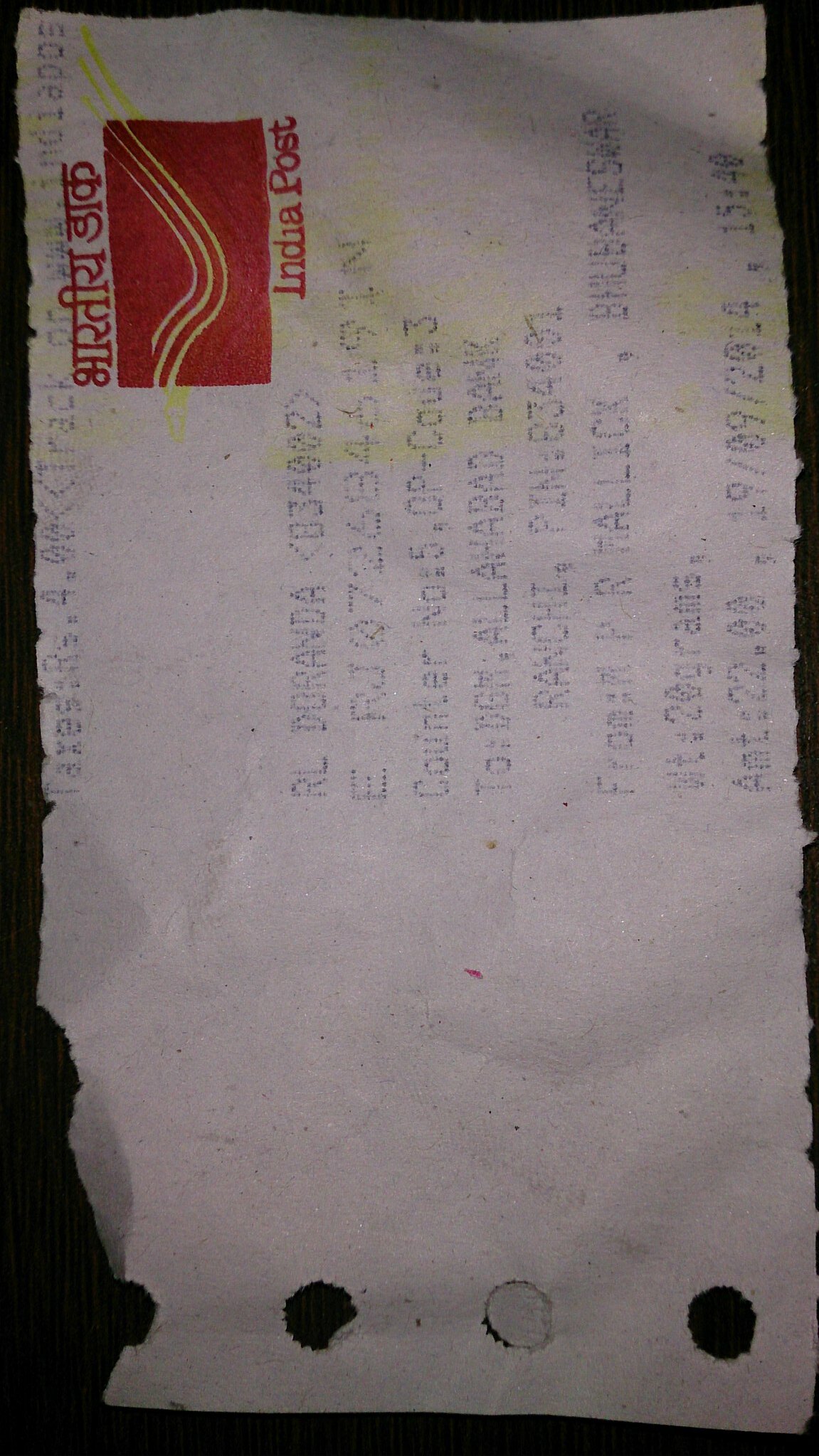The image features a white piece of paper that is slightly turned to the side, making the text on it somewhat difficult to read. The paper has three hole-punch holes along one edge, indicating it was torn from a binder or notebook. At the top of the paper, there is a red square logo with yellow, swirling lines running through it. Below the logo, the text reads "India Post." 

Further down the paper, part of the text is visible, showing segments such as "RL," "DOR ANDA," and the number "834002." Additional text includes the word "counter," followed by the number "two" and the abbreviation "PIN," indicating a PIN number. The arrangement and visible details suggest the paper might be a receipt, form, or piece of mail.